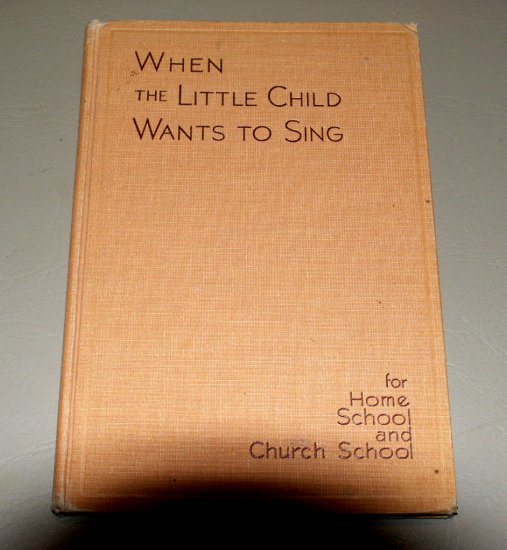The image showcases a worn, light tan book cover with a woven texture, lying on a gray background. The title on the book reads, "When the Little Child Wants to Sing," written in dark brown or gray lettering near the top. In the bottom right corner, it states, "For Homeschool and Church School." The cover appears aged, with slightly frayed corners, and it's unclear whether there is an actual book or journal inside. A half-circle shadow falls at the bottom of the image, adding depth, while light highlights the textured surface of the cover. Aside from these elements, the image is devoid of any other objects or text.